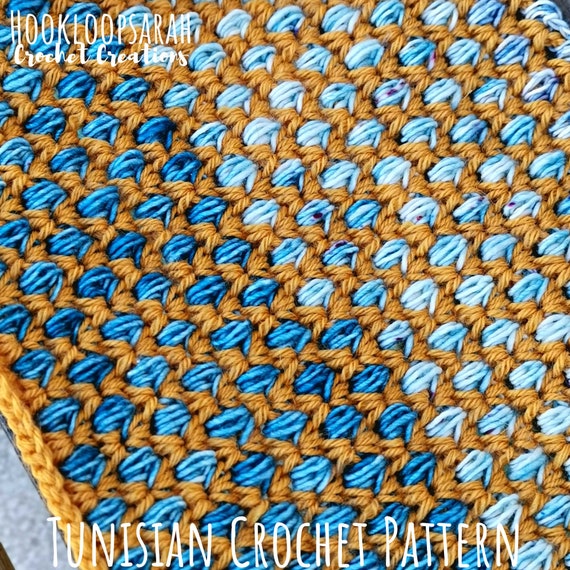The square image, approximately four inches by four inches, features an intricate Tunisian crochet pattern. Dominated by interwoven blue and brown threads, the pattern creates an appearance akin to a dull yellow fence set against a shifting blue sky. The top left corner showcases the text "HOOKLOOPSARAH" in all-caps white letters, followed by "crochet creations" in smaller, bold white cursive. The bottom of the image prominently displays "TUNISIAN CROCHET PATTERN" in tall, white capital letters. The pattern itself consists of five to six mostly parallel blue lines running from the top right to the bottom left, interspersed and bordered by brownish yarn that forms an X-shape with dark blue threads horizontally traversing the inside. The left half of the image is cast in shadow, while the right half is illuminated by sunlight, adding depth and contrast to the crochet design.